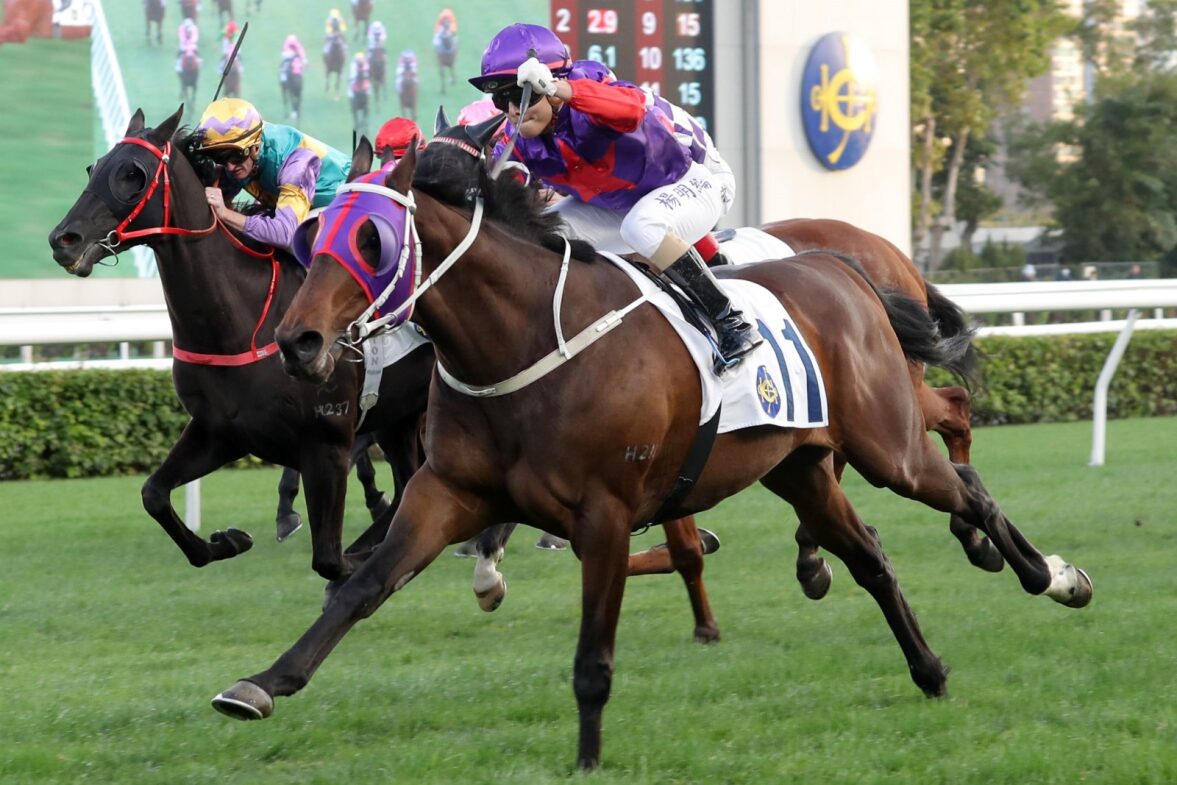In this detailed daytime photograph of a horse race, three racehorses are captured mid-race on a grassy track. The lead horse is dark brown with striking black legs, wearing a distinctive purple and red-striped mask with eye holes, connected to its jockey by white leather straps. This jockey dons a purple shirt with a red star, white breeches, black boots, and a purple helmet. The second horse, also dark brown, is partially visible, with only its rear end and the top of its jockey’s head showing. The third horse is black, ridden by a jockey in a yellow and purple hat, clad in a vibrant ensemble of green, yellow, and purple. Throughout the image, the riders sport bright and colorful attire, highlighting their gear's vivid hues and intricate patterns.

The grassy track is bordered by a white fence and lush green hedges, with a large screen in the background displaying an overhead view of the race, complete with numbers and logos. Surrounding the racecourse are vibrant green trees, adding to the lively atmosphere of the event. This photograph not only captures the intensity of the race but also the detailed preparations of both horses and jockeys, against a backdrop of well-maintained greenery and spectator amenities.